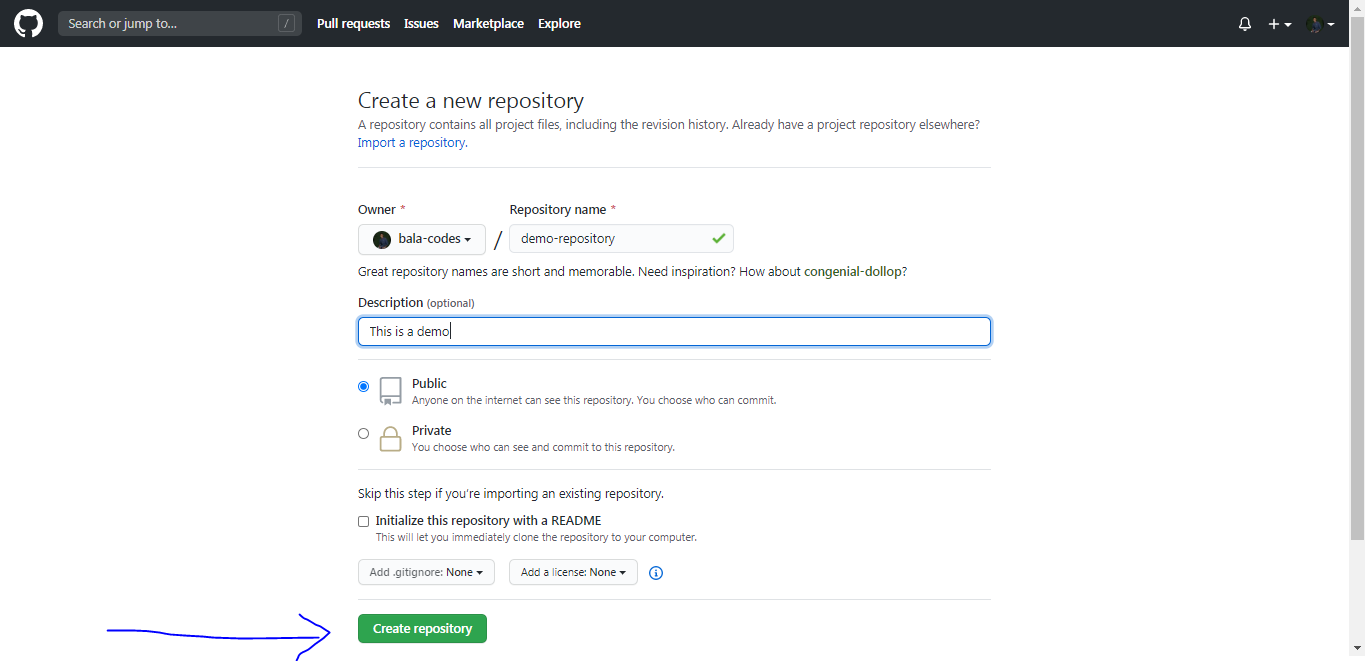The screenshot depicts a detailed view of a repository creation page on a code hosting platform, likely GitHub based on the layout and terminology. At the top of the page, there's a black navigation bar. On the left side of this bar, there is a white circle icon, possibly featuring a symbol that is hard to discern—it might be the silhouette of a person, a cat, or a tulip.

Next to the white circle, there is a search bar labeled "Search or jump to". To the right of this, several clickable options are visible including "Pull requests", "Issues", "Marketplace", and "Explore". Further along the bar are a bell icon for notifications and additional small icons representing plus and minus signs for potential configuration options.

In the main body of the page, centrally placed text reads "Create a new repository". Below this instruction, a brief description explains, "A repository contains all project files, including the original history. Already have a project repository elsewhere?" followed by a blue button saying "Import repository".

Below these descriptions is a form field labeled "Owner", with "Bala codes" selected. The next field is "Repository name", which has "demo repository" entered and is validated with a green check mark. A tip below these fields reads, "Great repository names are short and memorable," and offers a quirky suggestion, "Need inspiration? How about congenial dollop?"

The "Description" field is marked as optional, with the placeholder text saying, "This is a demo." Users can then choose the repository's visibility status, with "Public" selected and explained: "At public, anyone on the internet can see this repository. You choose who can commit." Alternatively, "Private" is briefly described: "You choose who can see and commit to this repository."

An optional step advises, "Skip this step if you're importing an existing repository." Additional options include a checkbox labeled "Initialize this repository with a README", to enable immediate local cloning.

Further configuration options include adding a `.gitignore` file or a license, both set to "none" by default. The form concludes with a prominent green button labeled "Create repository" in white text. A blue marker or arrow scribble points towards this button, indicating it as the final action to complete the process.